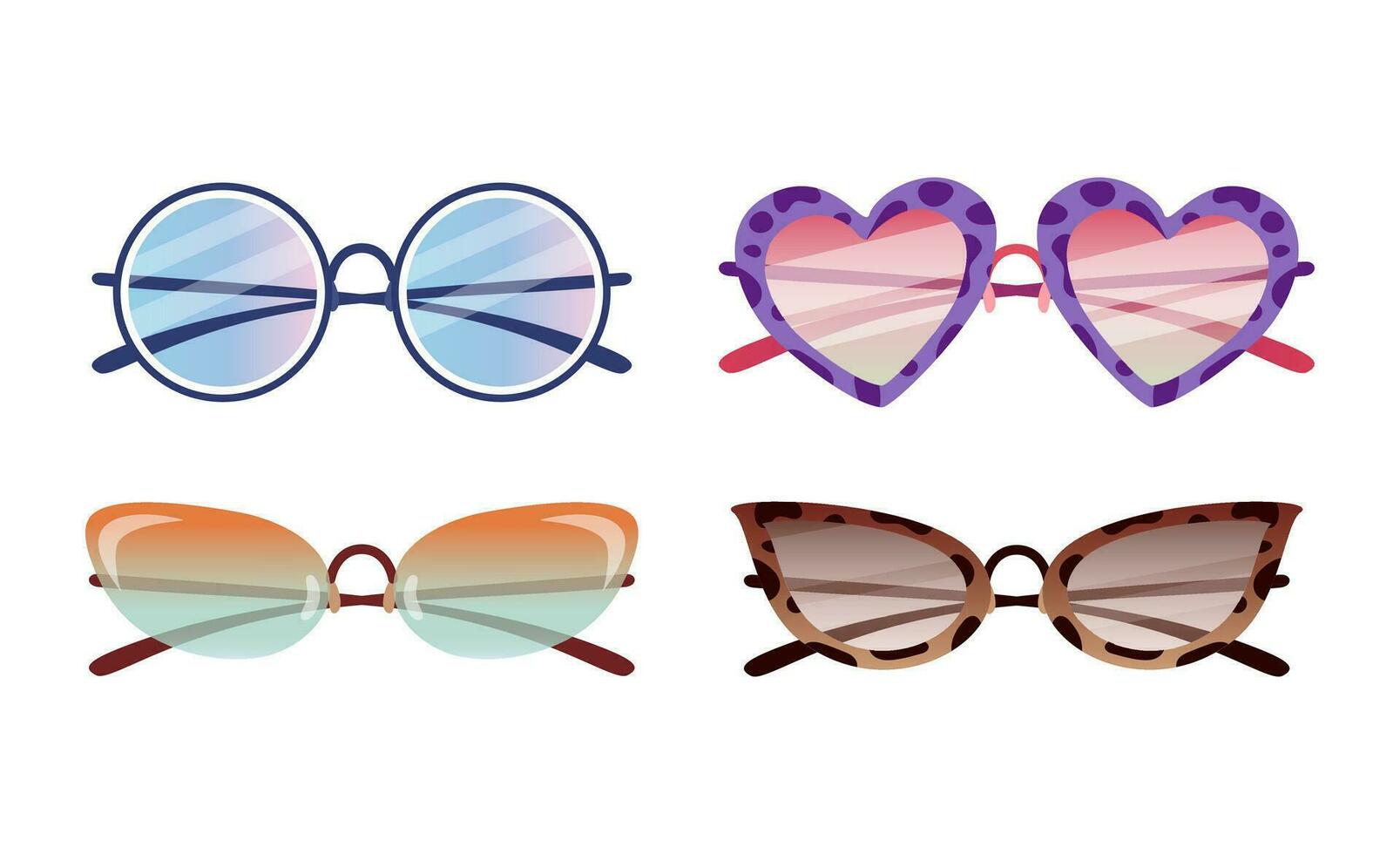The image is a color illustration of four distinct pairs of fashionable sunglasses arranged in two rows, two pairs on top and two on the bottom, set against a white, floating background. The top left corner features round sunglasses with a dark gray wireframe and blue lenses, with the arms folded inwards. To their right are heart-shaped sunglasses with a purple frame adorned with dark purple dots and pink arms. The bottom left showcases cat-eye rimless sunglasses that transition from aqua at the top to orange at the bottom. On the bottom right, there is another pair of cat-eye sunglasses with a frame in beige and black spots, and brown-tinted lenses. The overall style of the image is a vibrant and detailed color illustration, capturing a variety of eyeglass designs and colors.